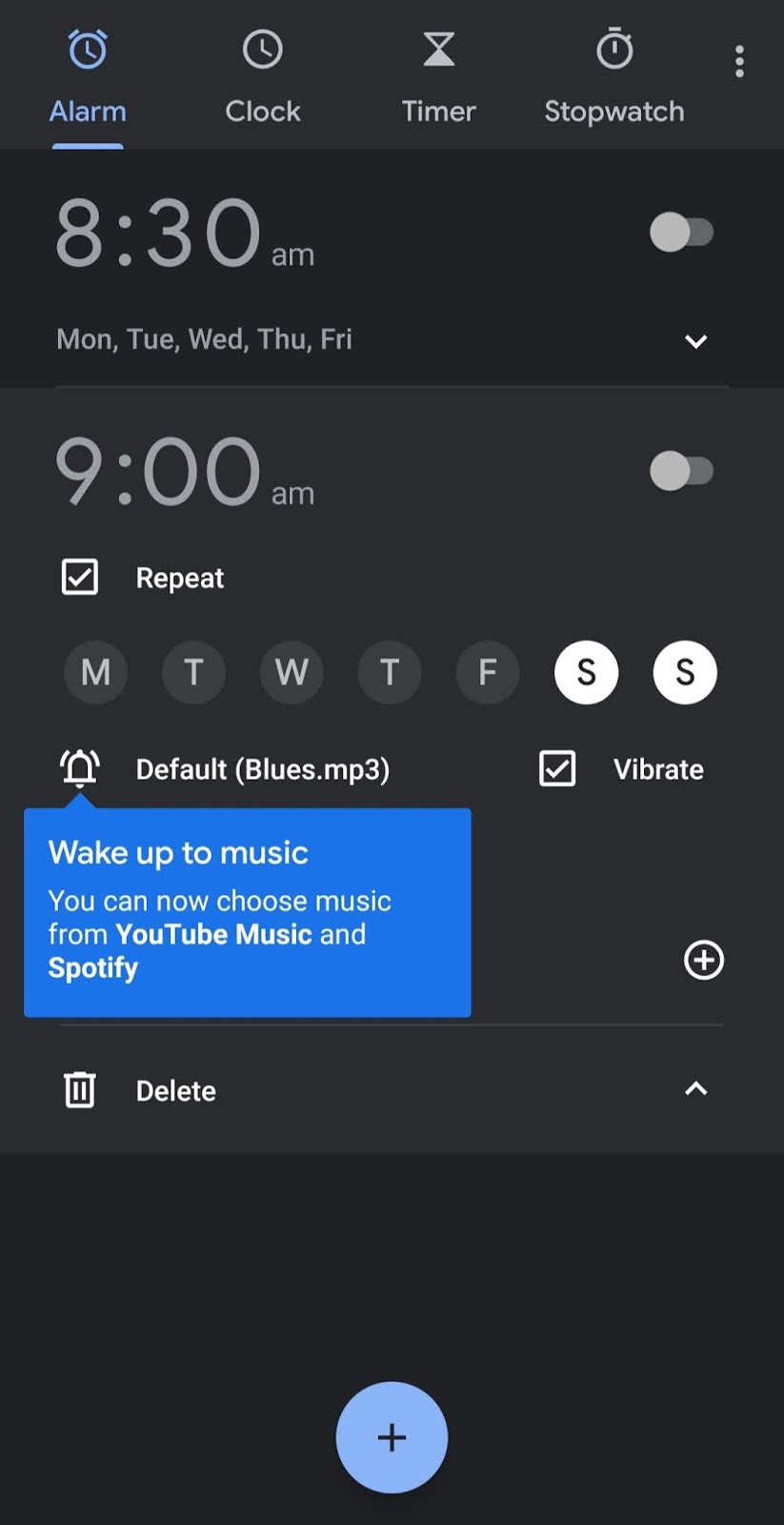The screenshot displays the Clock application on an Android cell phone, set against a solid black background. At the top of the screen, there are four horizontally aligned icons typical for Android clock apps: an active blue alarm icon on the left, followed by a clock icon labeled "Clock," a timer icon labeled "Timer," and a stopwatch icon labeled "Stopwatch" on the far right.

Below the top icons, two alarms are set but currently deactivated. The first alarm is set for 8:30 a.m. on weekdays (Monday through Friday) and features a checked "Vibrate" option. The second alarm is set for 9:00 a.m. on weekends (Saturday and Sunday), also with the "Vibrate" option checked.

Further down, beneath a notification bell icon, the selected alarm tone is indicated as "default_blues.mp3." There is a prominent blue box below this information, featuring a message in white lettering: "Wake up to music. You can now choose music from YouTube Music and Spotify." On the right-hand side of this box is a plus icon, allowing users to add their own tone. Beneath the blue box, a white trash can icon labeled "Delete" provides an option to remove alarms. 

At the bottom of the screen, a blue circle with a black plus sign at its center offers a straightforward means to add new alarms.